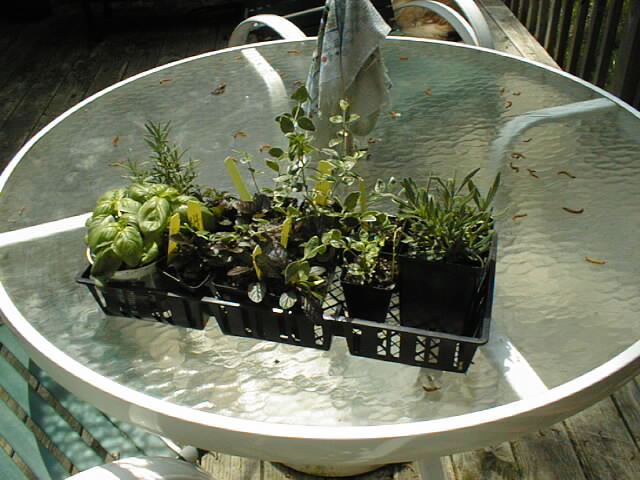This image depicts an outdoor scene on someone's wooden deck, focusing on a glass-topped patio table with a white frame. On the table, there is a black tray holding several small black containers, each containing a variety of green, leafy plants, likely part of a plant starter kit for herbs such as basil, rosemary, thyme, and mint. The plants differ in appearance; some are broader and wider, others are pointy or vine-like. Scattered around the tray are brown, dried leaves. Below the table, you can spot two green and white chairs, and a piece of a blue item, possibly part of a chair. In the background, a wooden fence frames the area, suggesting it is an enclosed space.